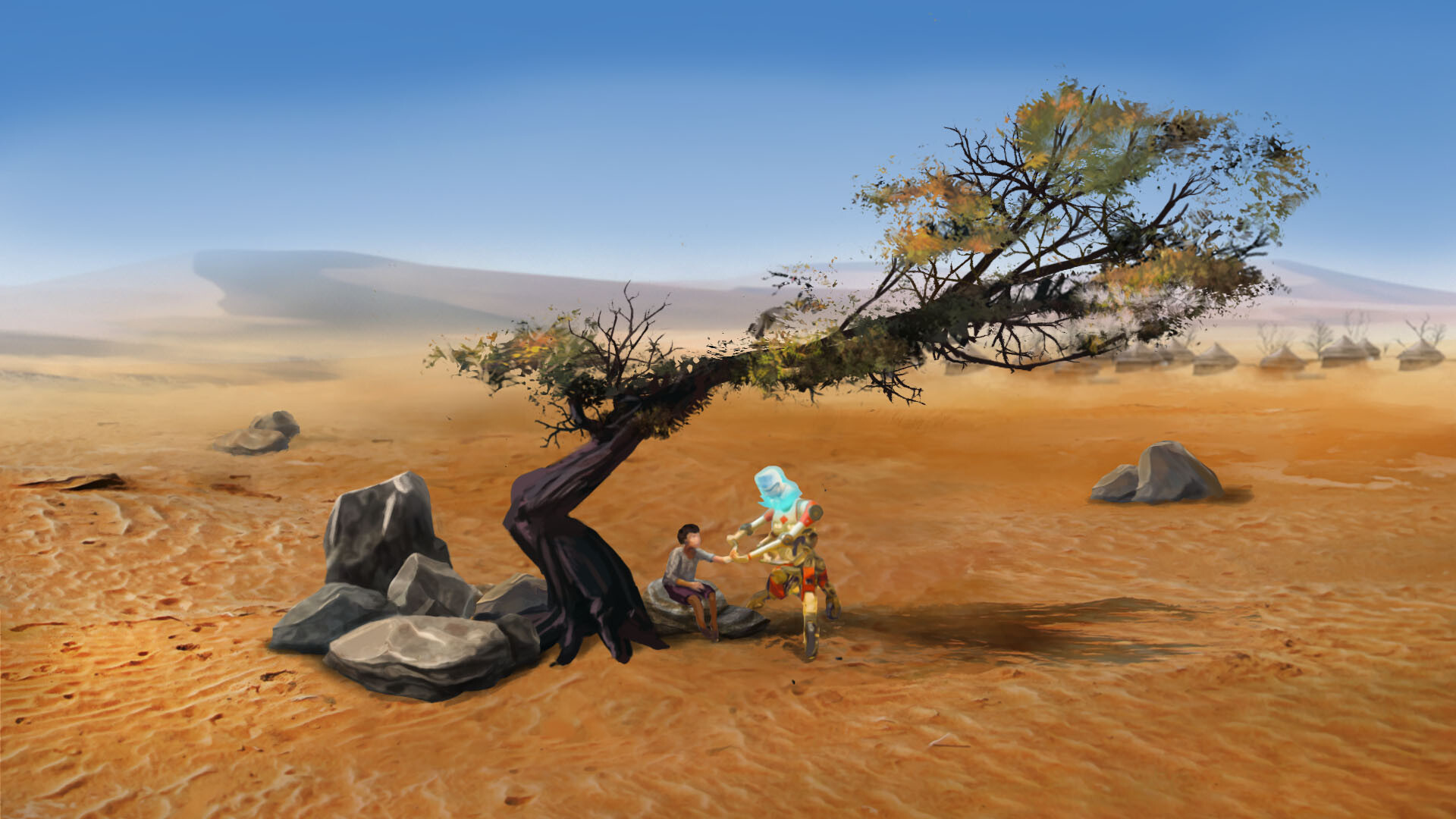The digital print depicts a surreal desert landscape with rolling sand dunes and distant hills under a clear blue sky with the slightest hint of mist-like clouds. Dominating the foreground, a peculiar tree with branches extending horizontally emerges from the sandy ground. Located just left of center, this tree is surrounded by an arrangement of five gray boulders, with more scattered rocks and unusual, dome-shaped buildings visible in the background on the right.

Beneath the tree's sparse shade, a young boy sits on a boulder, engaged with a robot. The robot, which features a human-like head shrouded inexplicably in a blue covering, has three legs and two arms, one of which is gently interacting with the boy's hand. In the background, additional trees with similarly bizarre forms and approximately ten to twelve dome-shaped structures contribute to the setting's otherworldly feel. The color palette primarily consists of earthy tones—tan, brown, light brown—interspersed with soft greens, grays, and varied shades of blue, emphasizing the barren yet strangely captivating environment.